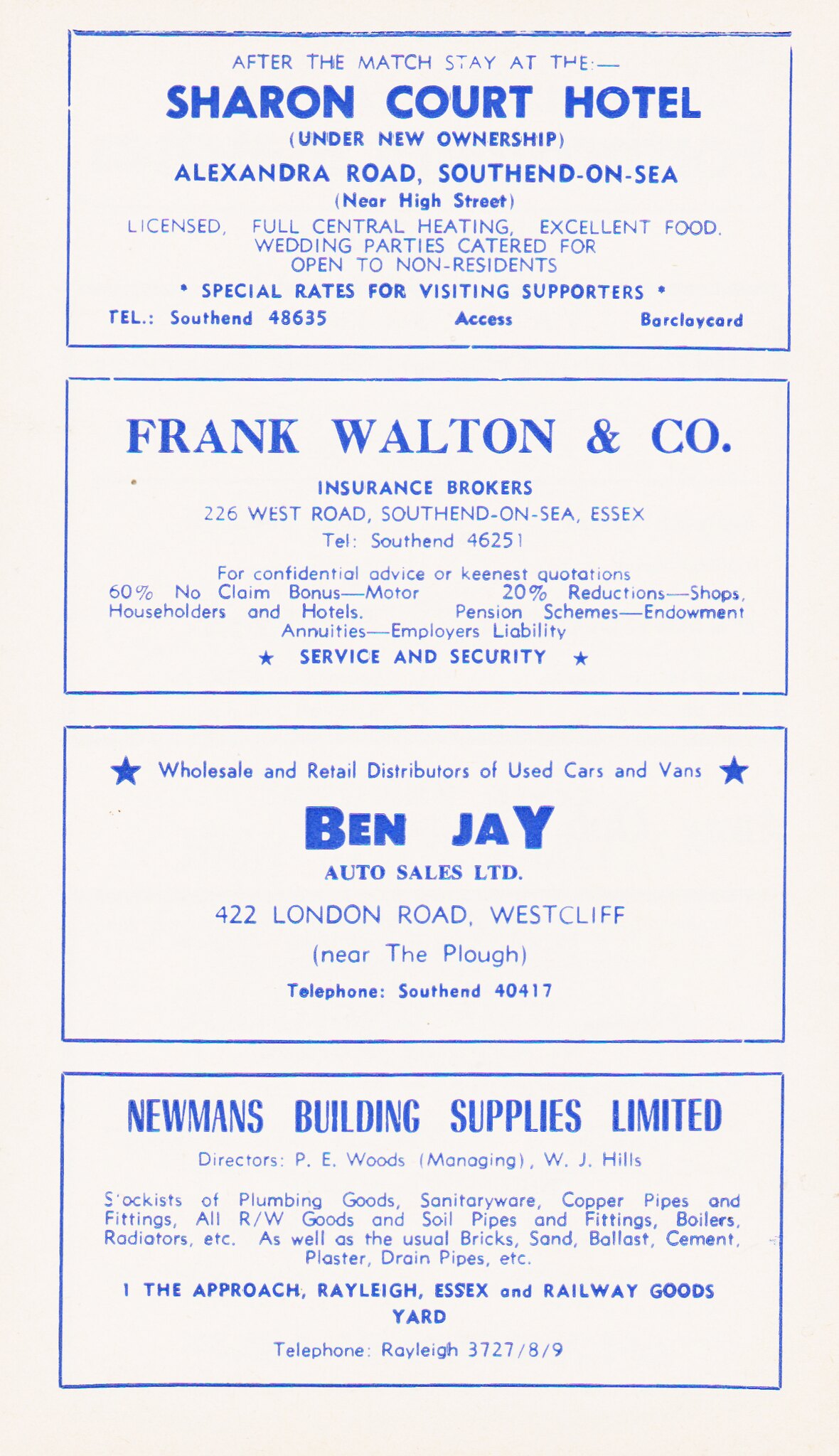The image features a vintage advertisement comprised of four stacked blue rectangles resembling business cards, each with detailed information in blue font. The first rectangle promotes the Sharon Court Hotel on Alexandra Road, South End on Sea, offering special rates for visiting supporters with amenities like central heating and excellent food; it mentions being under new ownership. The second rectangle displays Frank Walton and Company, Insurance Brokers, located at 226 West Road, South End on Sea, Essex, emphasizing "service and security." The third rectangle advertises Ben J, Auto Sales Ltd, wholesale and retail distributors of used cars and vans, situated at 422 London Road, Westcliff, near the Plough pub, complete with a telephone number. The final rectangle showcases Newman's Building Supplies Limited, managed by Directors P.E. Woods and W.J. Hills, offering plumbing goods, sanitary ware, copper pipes, and fittings; located at The Approach, Raleigh, Essex, and Railway Goods Yard, including a contact telephone number. Each rectangle utilizes blue rectangles as a backdrop for the text, giving the advertisement a cohesive look.